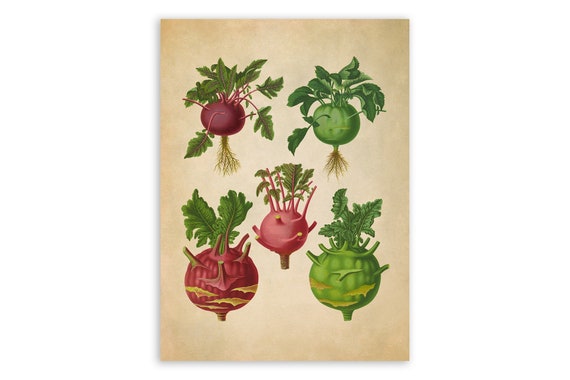This botanical illustration captures a variety of radishes, meticulously detailed to showcase their diversity. At the upper left, a traditional red radish is depicted with leafy green tops and visible roots extending beneath. Adjacent in the upper right, a unique green radish stands out, characterized by its vibrant color and similar leafy and root structure. The central radish, familiar from grocery stores, displays modest leaves and minimal roots, presenting a pinkish hue. In the lower left, a large, round radish features vertical striations and a purplish-red tone, with sprouts emerging prominently. The lower right radish, comparable in size to its neighbor, intrigues with its green coloring and subtle detailing. Notably, the illustration's style, reminiscent of watercolor on aged paper, imbues the radishes with a timeless, artistic quality.